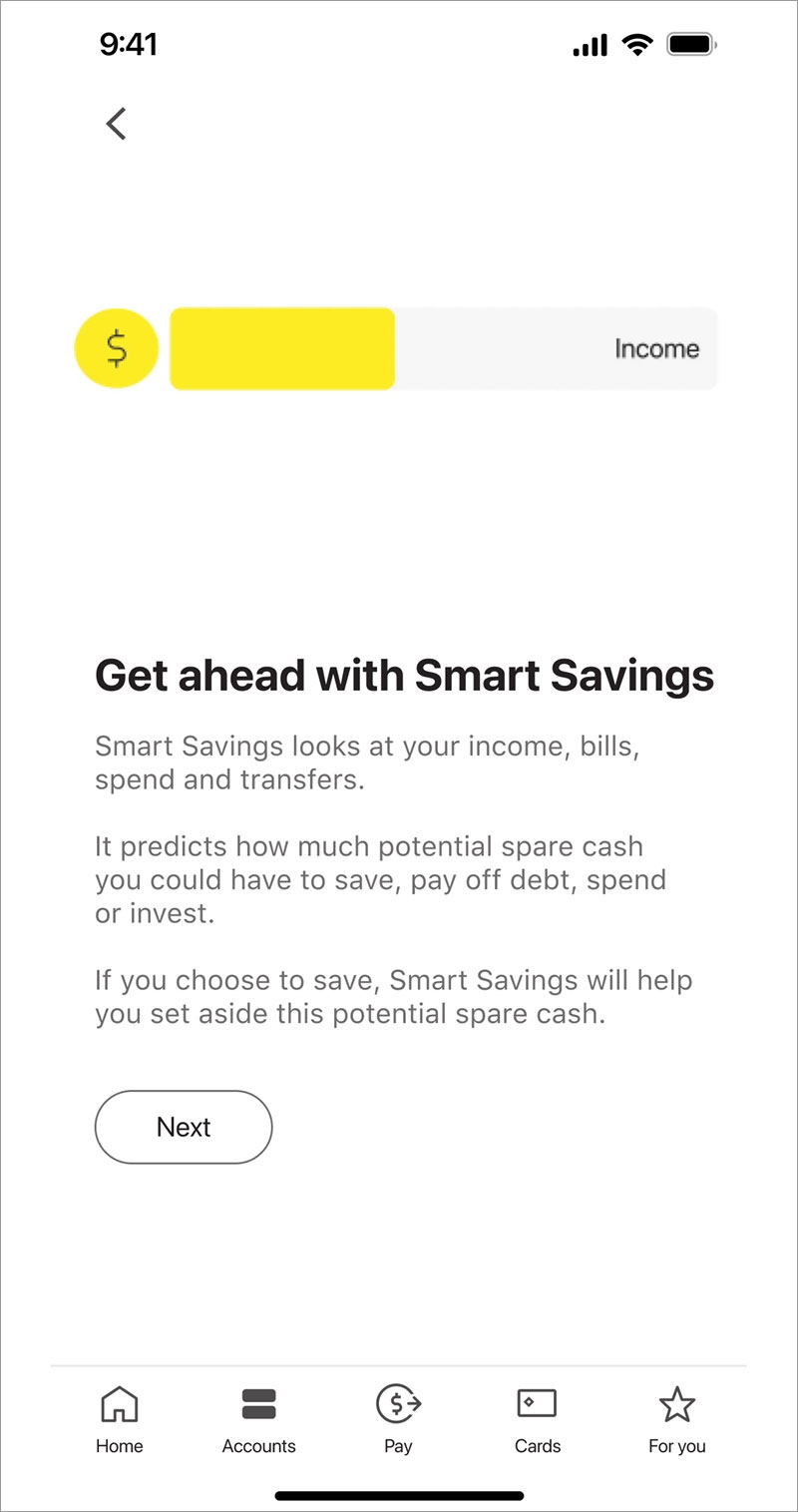The screenshot displays a financial savings interface on an iPhone, as identified by the icons at the top of the screen. At the upper left corner, there is a left-facing arrow, likely intended for navigation to a previous page. Below this, a vibrant bar chart appraises the page with the only touch of color. This chart depicts 'Income,' with an accompanying yellow circle featuring a dollar sign on the left. The progress bar extends to the right, demonstrating that approximately 40-45% of the bar is filled in bright yellow, symbolizing earned income, while the remaining 55-60% is grey, indicating a portion yet to be allocated.

Following the bar, informative text reads: "Get ahead with Smart Savings. Smart Savings looks at your income, bills, spend and transfers. It predicts how much potential spare cash you could have to save, pay off debt, spend or invest. If you choose to save, Smart Savings will help you set aside this potential spare cash." Beneath this description, a "Next" button invites the user to proceed.

Finally, the bottom of the screen features navigation icons for actions such as home, accounts, pay, cards, and a personalized section labeled "For You," providing quick access to other functionalities of the application.